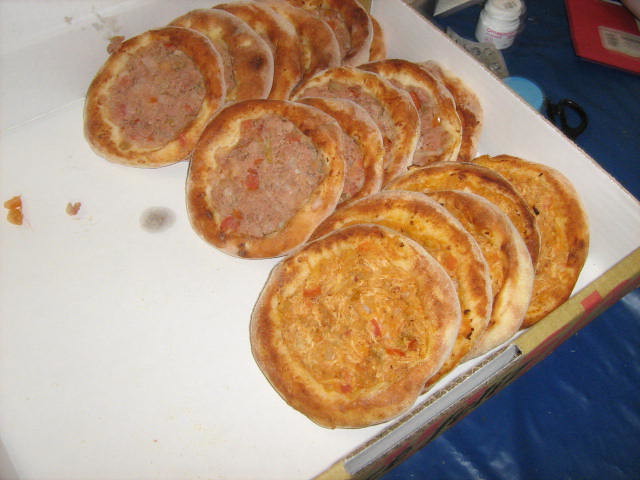The image features a partially open white cardboard box, approximately half-full with neatly stacked round pastries, resembling small tarts or dough rings filled with a savory meat substance and possibly bits of reddish tomato-like elements. Each pastry boasts a golden-brown crust, positioned on their sides to form rows within the box. A noticeable grease stain marks the center of the box, alongside scattered pastry flakes. The box rests on a white table that has a brown edge, ensuring the pastries stay contained. Out of focus in the background, the blue and white mottled tile floor holds various small objects, including a pill bottle, a red envelope, and other miscellaneous items. The overall scene captures the detailed textures and arrangement of the pastries against the contrasting backdrop.